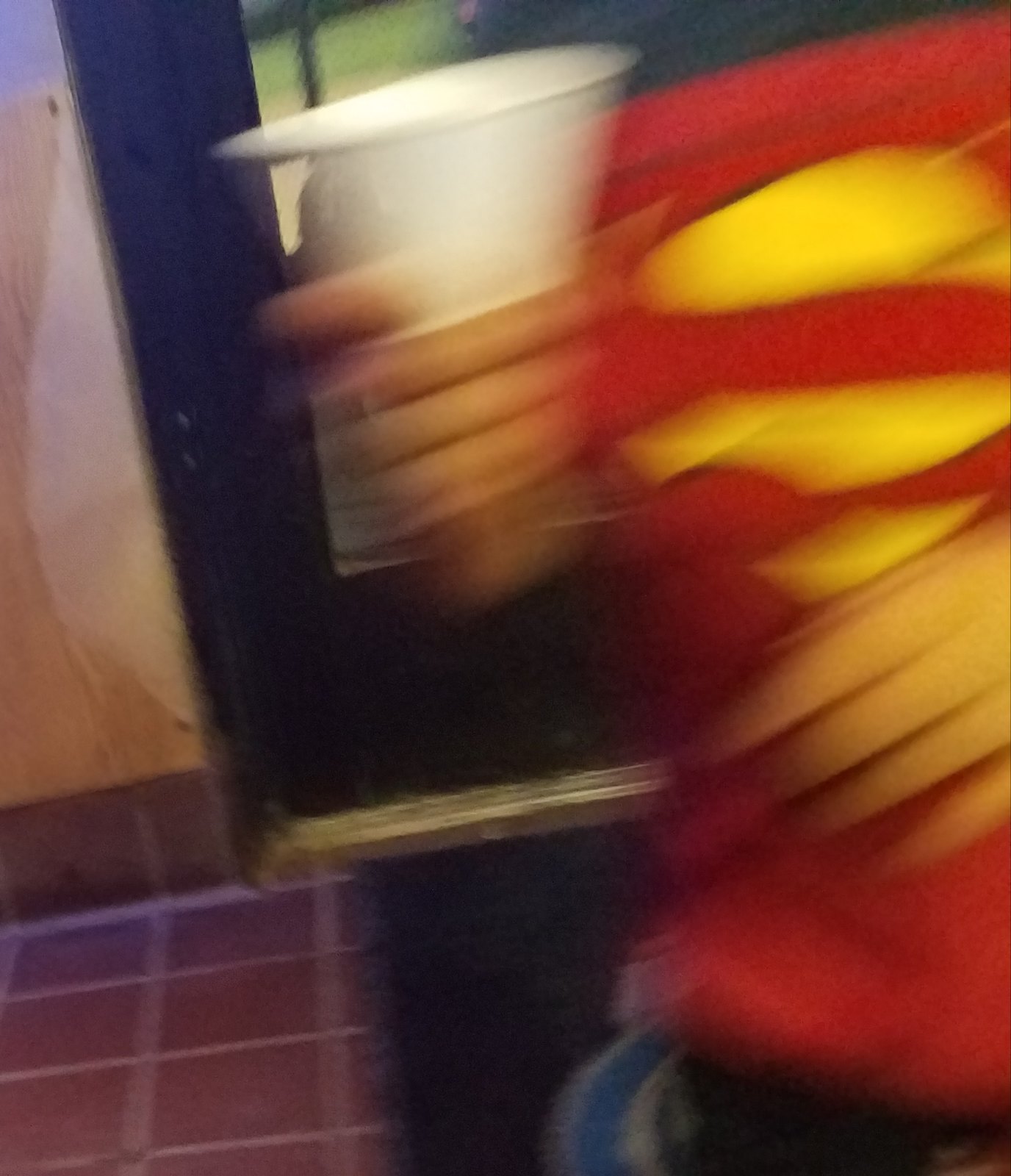In this blurred, portrait-oriented photograph, we see a Caucasian individual standing against a background that includes a brown-tiled floor and a wooden wall rising up from it. The person is captured from chest level to the top of their right thigh, with their head and lower body out of frame. They are donning a short-sleeved, red Superman t-shirt with a yellow 'S' logo that appears intentionally distressed, as if the red surface has been artistically scratched to reveal the emblem beneath. In their right hand, they hold a white paper cup, presumably filled with a beverage, likely obtained from a black machine behind them. This context suggests the setting might be a cafe or restaurant. The person is positioned towards the right side of the frame, facing the viewer with their torso, while turning away from the machine, possibly heading back to a table.